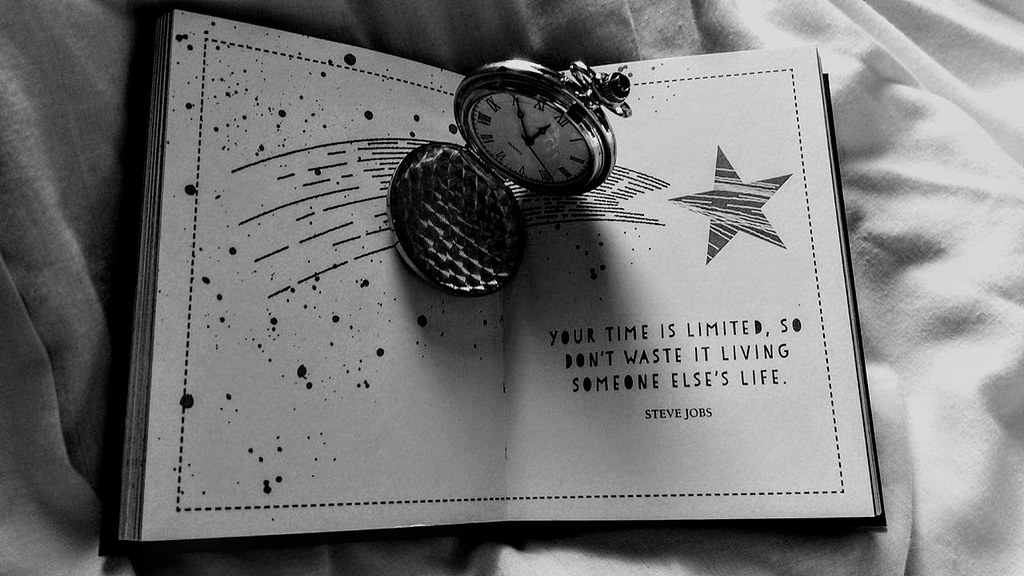This black and white photograph captures an open book resting on a soft, light-colored blanket. A small, open pocket watch sits precisely in the center of the book's crease, displaying a time close to 10 minutes to 12. The left page of the book features an artistic design of paint splatters and broken lines, transitioning into the continuous tail of a comet that elegantly arches across to the right page. On the right page, bold black text reads, "YOUR TIME IS LIMITED, SO DON'T WASTE IT LIVING SOMEONE ELSE'S LIFE," attributed to Steve Jobs. This evocative image combines art and a poignant quote to convey a powerful message about the value of time.